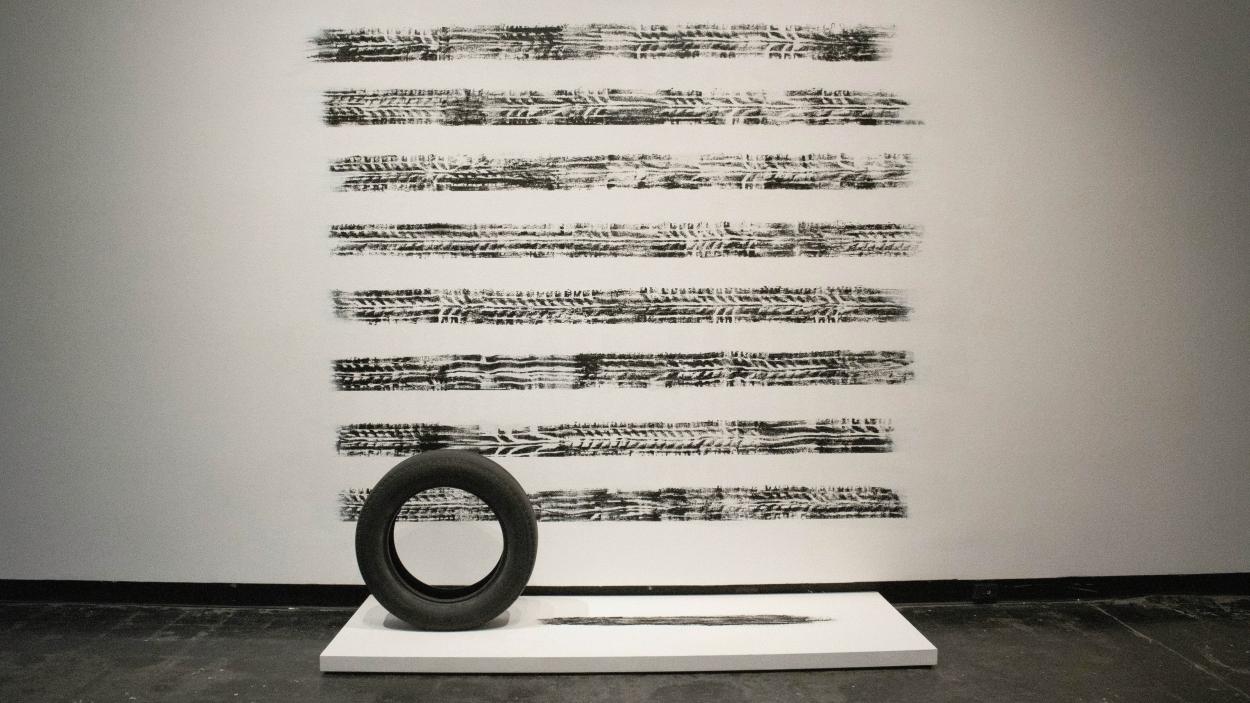The photograph captures an abstract art installation in an art gallery. At the center of the setup is a low white platform, a couple of inches high, set against a light gray or white wall and a dark black floor. On the left side of the platform, an upright black car tire is prominently displayed. Adjacent to it, extending to the right and covering about three-quarters of the platform, is a painted black tire track. Above this arrangement, the wall features eight horizontal bands of black tire tracks, creating a unique display of patterns in ink or paint.